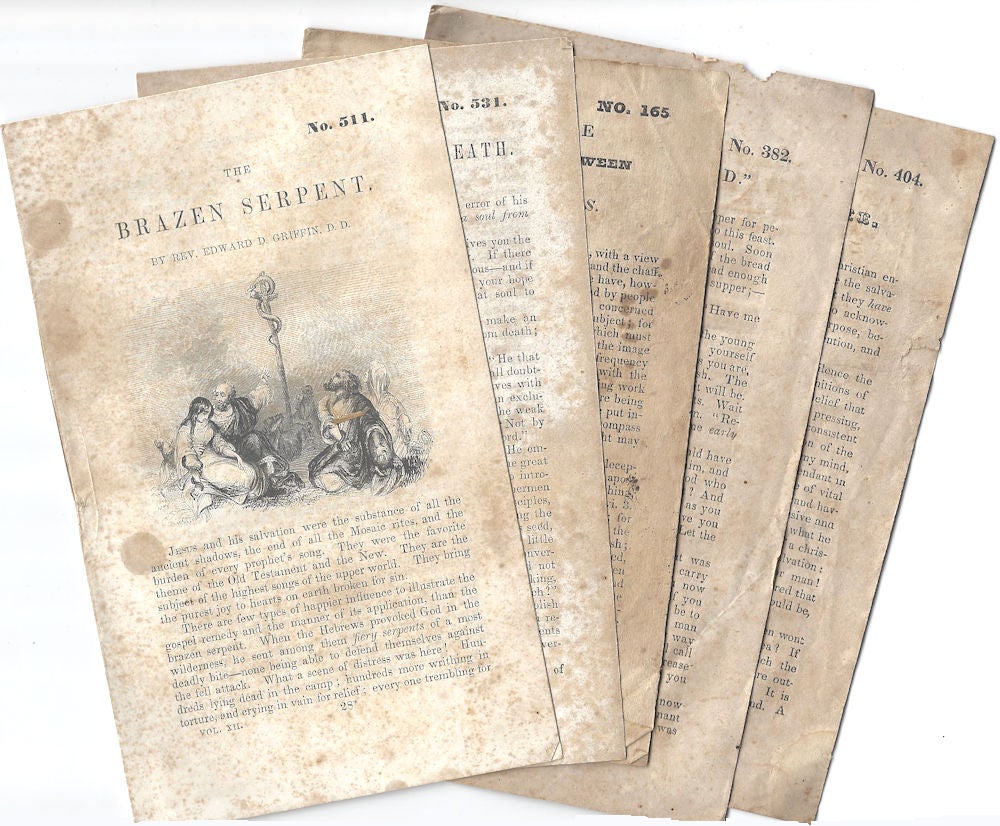The image depicts five aged, brown, and oxidized pages that have been torn from a book, likely historical or religious, as indicated by their appearance and content. These pages, frayed and stained, are arranged in a slightly fanned-out manner, overlapping each other and partially obstructing the view of the text on some of them. Each page is numbered in the top right corner, with the numbers being 511, 531, 165, 382, and 404. 

The first page, labeled as number 511, features prominently and is the most detailed. The title at the top reads "The Brazen Serpent" by Rev. Edward D. Griffin, D.D. Below the title, there is a faded black-and-white illustration showing a scene where an elderly man with a beard is seated and consoling a woman with long hair, both dressed in robes. They are surrounded by other people, some of whom are engaged in what appears to be prayer, and there is a staff with a snake coiled around it extending into the sky, depicted in the background of the image. This illustration is positioned above several paragraphs of text, though the specifics of the text are blurred and difficult to read due to the age and condition of the pages.

The font varies slightly between each page, with some featuring small, bold type while others have wider bold or normal styles, contributing to the distinct historical feel of the documents. The pages collectively present a glimpse into an ancient text, rich with detailed illustrations and narratives, indicative of their considerable age and possibly significant historical or religious value.